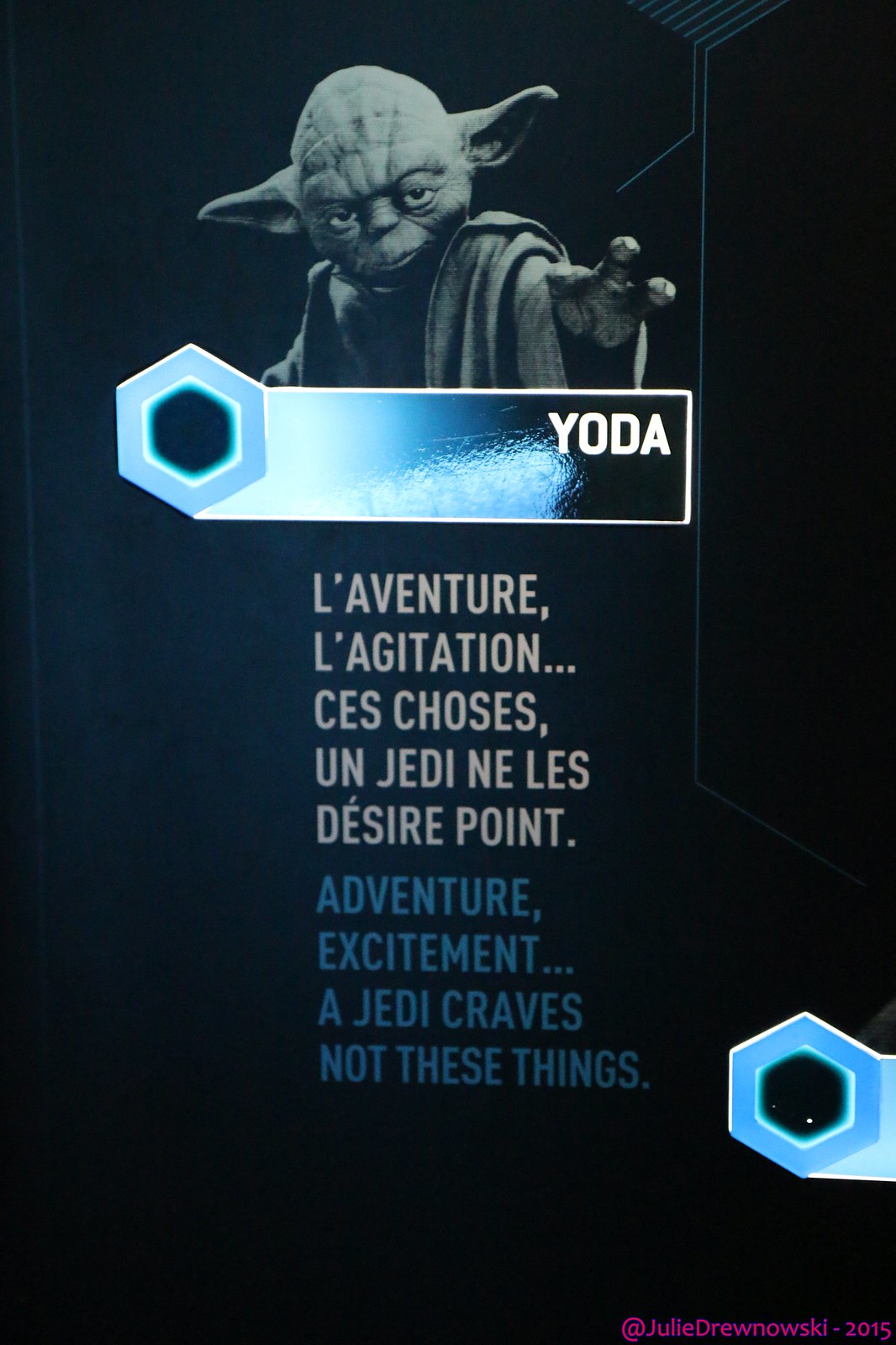The image is a vertically cropped photograph, likely a screen capture from a video game or some video, taken with a smartphone. It features the iconic Star Wars character, Yoda, from the chest up, set against a black background. Yoda, characterized by his green, frog-like face with large ears and a bald head, appears in a dark greenish, almost grayish tone. He looks very serious, staring intensely at the center of the image, with one hand up and three fingers pointed outward, while his other hand is obscured at the bottom, casting a shadow.

The image includes a graphic with a honeycomb design and the name "Yoda" in white font near the top center. Below it, five lines of French text in white read: "L'Aventure, L'Excitation, Ces Choses, Un Jedi Ne Les Désire Pas," followed by an English translation in light blue font: "Adventure, Excitement, A Jedi Craves Not These Things." Another honeycomb design in light blue with a black center appears at the bottom right, next to the credit "at Julie Dronowski 2015" in hot pink.